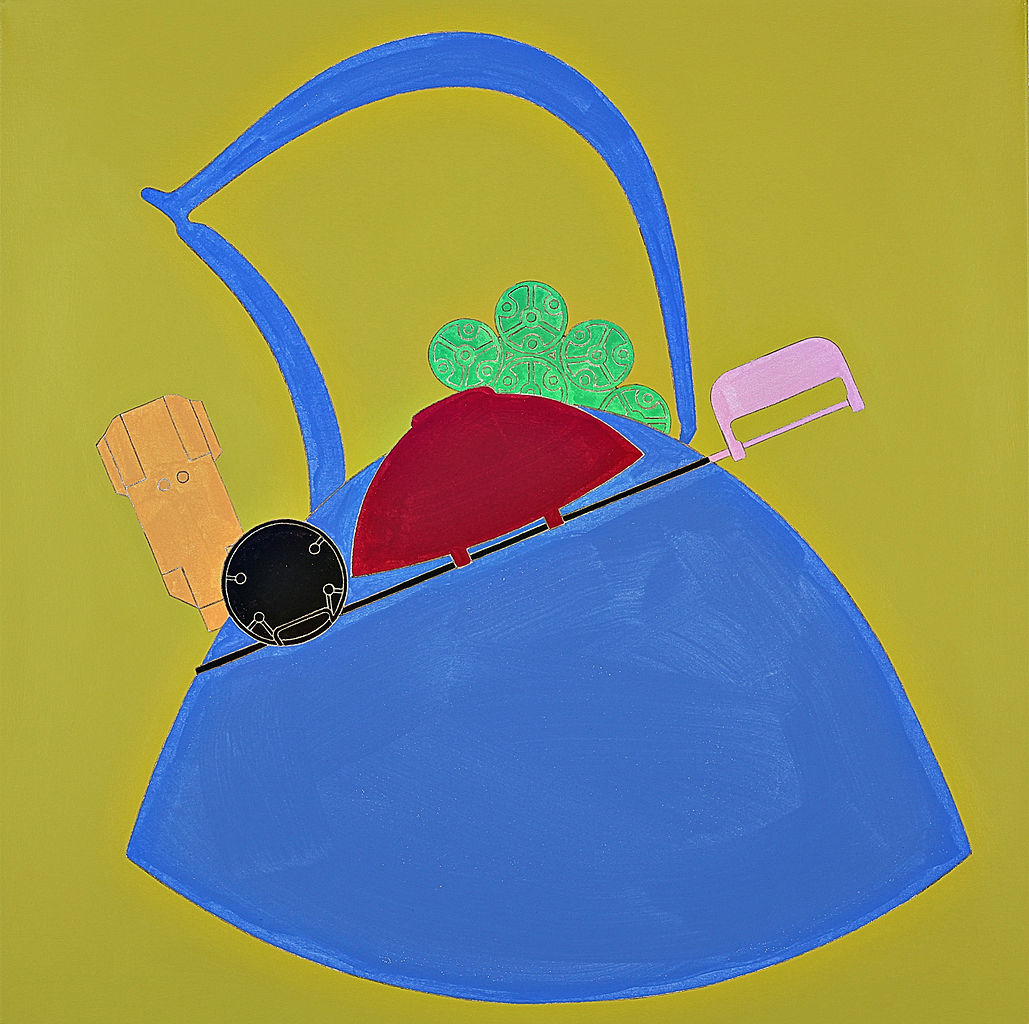This image is a vibrant, multi-colored painting against a mustard yellow background, predominantly featuring shades of blue alongside red, black, orange, green, and pink. At the center, there is a deep blue object that resembles a tea kettle or an old iron with a large, thin handle on top. Across the top of the kettle/iron is an abstract depiction of a needle or sword with a pink handle, holding an inverted red teacup or bowl and a round, black circular item at its end. Emerging from the back of the kettle/iron is an orange-toned, rectangular object, adding to the composition's intrigue. Surrounding the central object are five green circles, resembling either bubbles or leaves, contributing to the overall abstract nature of the painting.